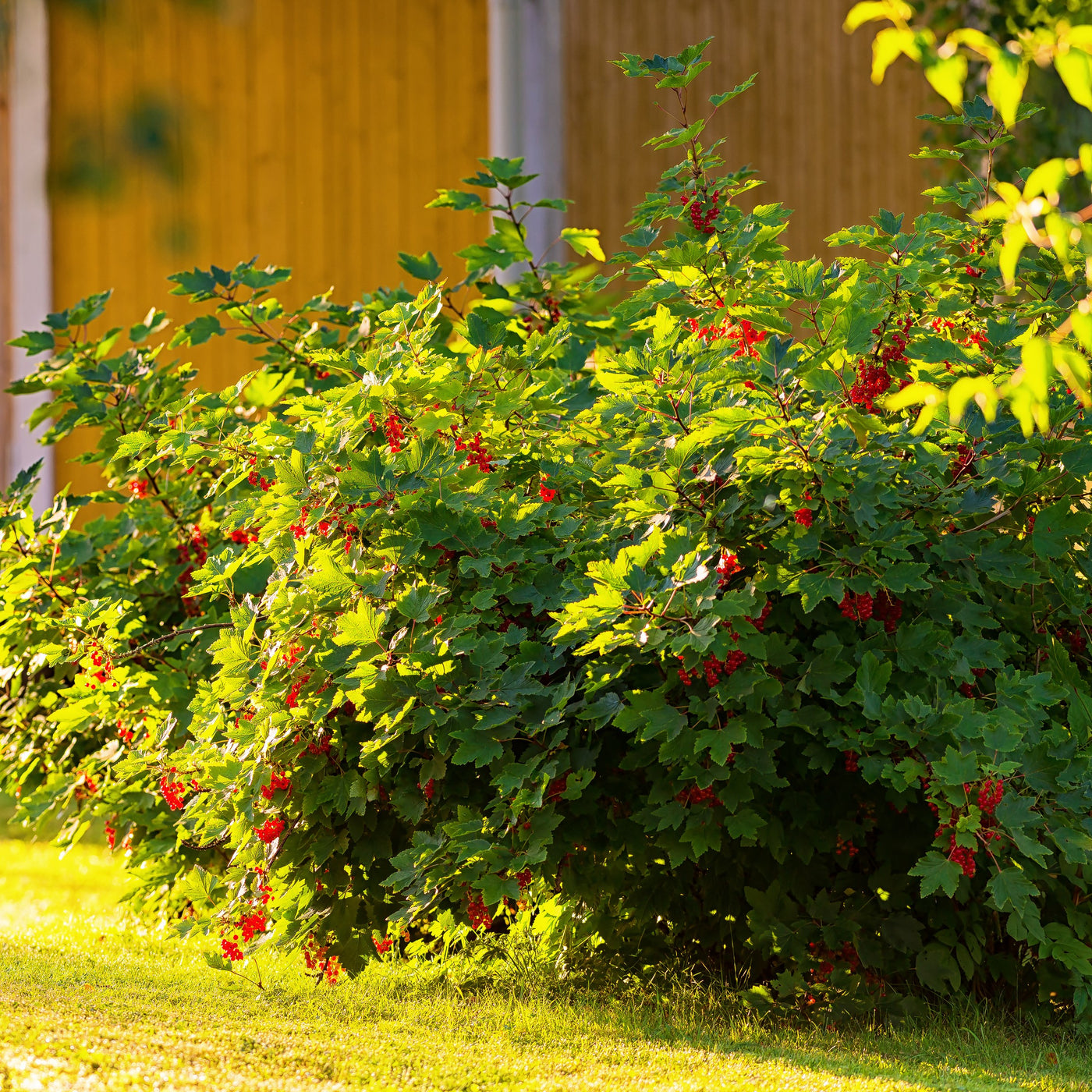The image captures a close-up of a lush bush with abundant green leaves interspersed with bright red flowers and berry-like fruits. The bush is situated adjacent to a wooden fence that varies in hue from light yellow-brown to light brown, with textures of vertical stripes made by the wooden planks. The fence also includes some gray posts that can be seen intermittently. Below the bush, the grass is a blend of light green and yellowish tones, likely due to sunlight filtering through. The light creates a striking contrast, with the top left of the image being brightly lit by the sun, while the bottom right appears more shaded. In the blurry top right corner of the image, a different type of plant can be seen. The photograph beautifully blends natural elements with a rustic wooden backdrop, highlighting the vibrant coexistence of flora and sunlight.